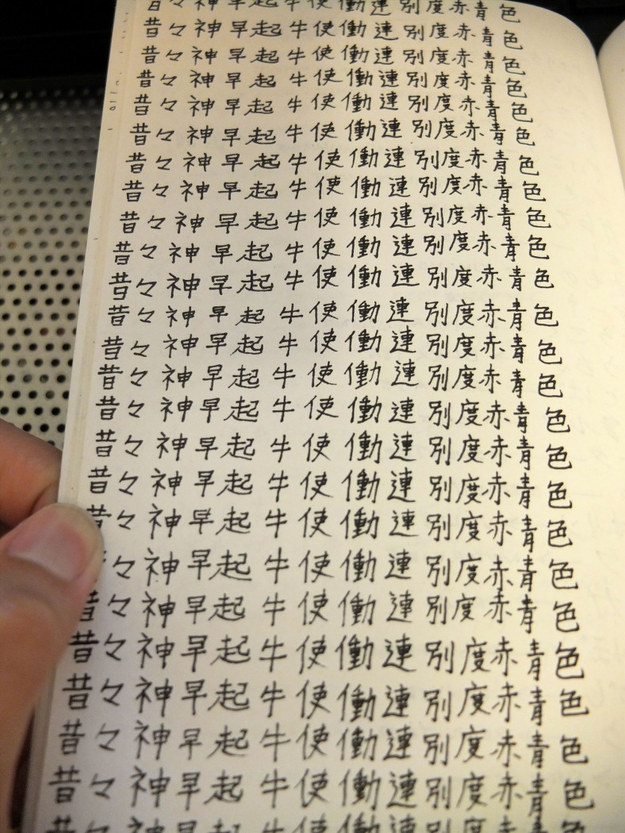This indoor photograph prominently features a hand, likely belonging to a person of non-brown complexion, holding a page from a book between the thumb and forefinger. The primary focus is the piece of paper covered in Chinese characters, arranged in roughly 15 vertical columns, each containing about 15 identical characters. The background, a gray and off-white polka-dot pattern, probably a tablecloth or wall, contrasts the tan, pink, white, black tones of the central image. The paper, resembling a narrow, receipt-sized strip, fills the majority of the frame, while the hand holding it is visible in the bottom left corner. The image closely captures the details of the characters, emphasizing their repetitive nature and ensuring no other text is present.